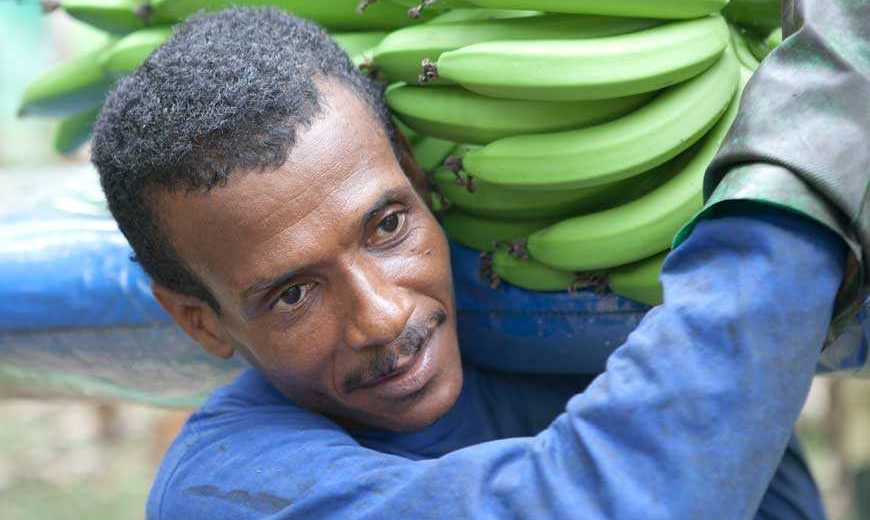The image depicts an African-American man with a receding hairline, short black hair, and a neatly trimmed mustache. He is wearing a long-sleeved blue shirt and black rubber gloves with green accents. He appears to be in an outdoor setting, as indicated by the background featuring a blue tarp. The man is carrying a large bunch of unripe, bright green bananas on his shoulder, using a blue pad for support. The ends of the bananas are brown, contrasting with the green fruit. His facial expression conveys a sense of weariness, suggesting he is experienced in physically demanding labor.